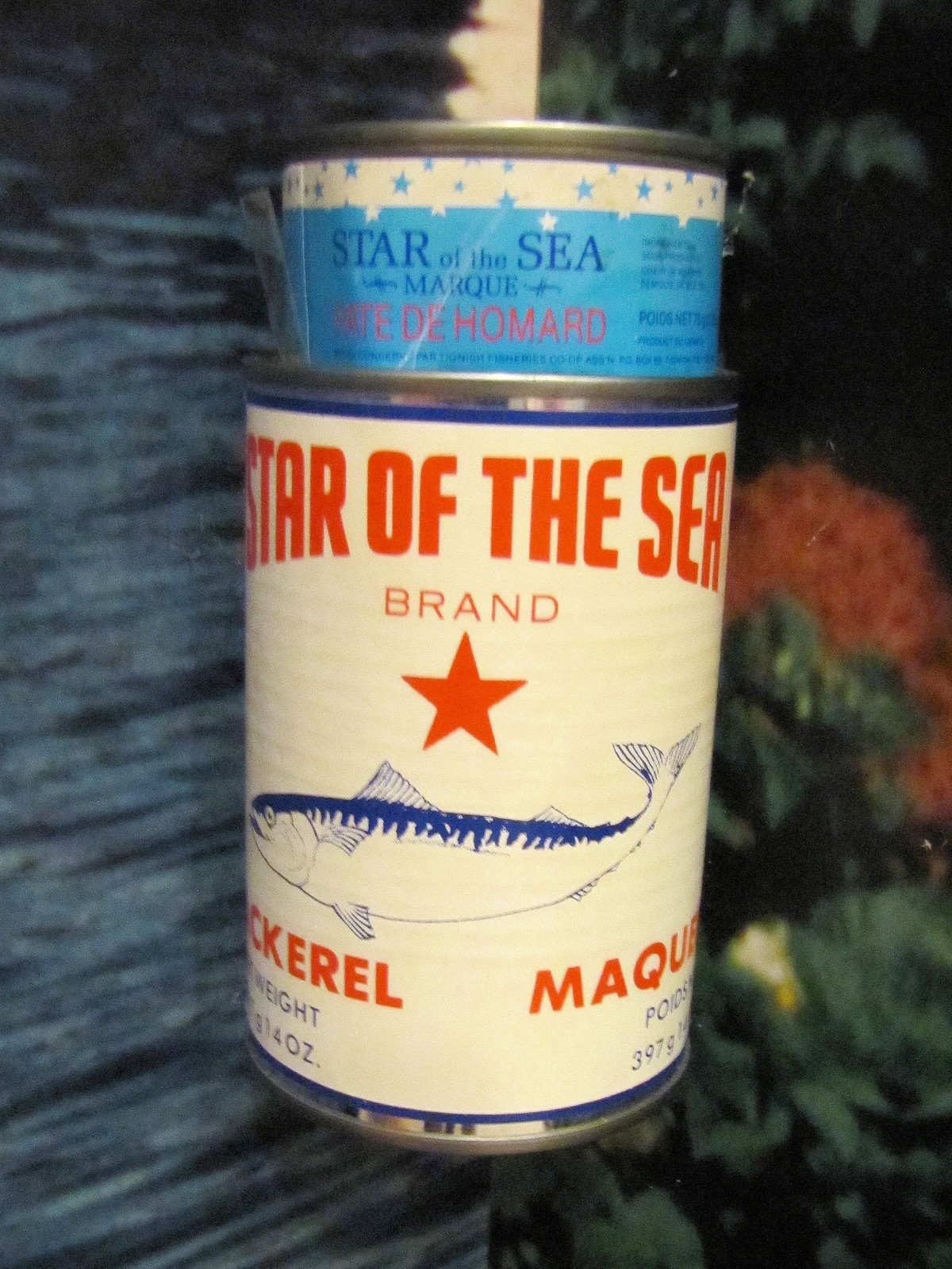In the image, two cans of fish are stacked on top of one another amidst a background of flowers or greens. The smaller top can is a half-height, blue-gray can with a predominantly blue label. This label features a white strip at the top adorned with blue stars, and reads "Star of the Sea" and "Marque" in French. Additionally, it says "pate de homard" in red text, indicating it contains lobster pate. The larger bottom can, roughly the size of a regular soup can, has a white background with red text. At the top, it boldly states "Star of the Sea Brand" followed by a prominent red five-point star. Below the star, there's a detailed blue illustration of a mackerel, and the word "mackerel" is written in red at the bottom of the label, along with a weight description in blue text.